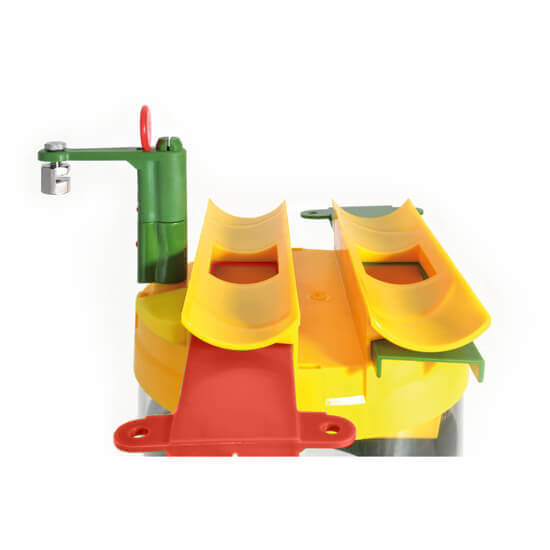This image showcases a close-up of an intricate, multicolored plastic toy. Dominating the scene is a yellow circular base adorned with two curved yellow rectangle pieces featuring square openings at the center. The left side of the toy presents a green 90-degree angle plastic piece, resembling a handle, topped with a red plastic disc and an attached hanging metal dial. Beneath the left curved rectangle is a red retractable pillar that can slide in and out, akin to a drawer mechanism but without a base. On the right, another retractable pillar in green mirrors this structure, though it lacks handles. A spout-like structure with a red turnable knob is situated on the far left. The toy's components, primarily green, yellow, and red, form a complex yet visually engaging device that's challenging to identify but appears to be made solely of plastic.